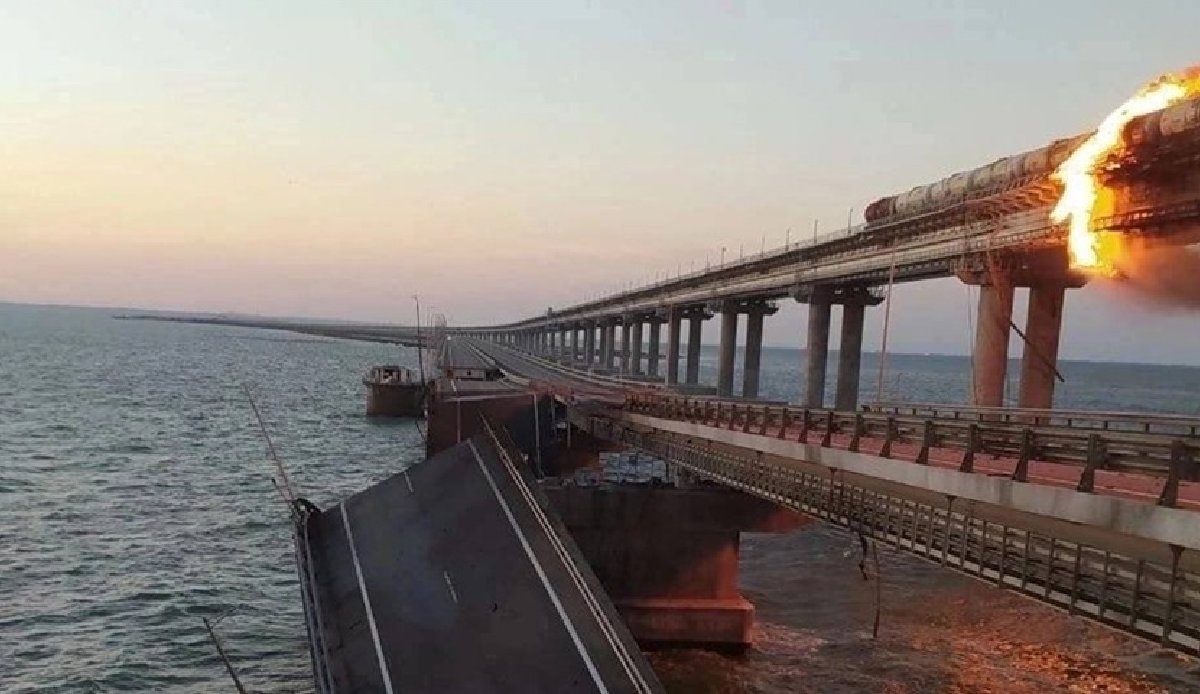The image captures a dramatic scene of a bridge set across a large, still body of blue water, possibly an ocean, with a striking sky that fades from gray at the top to light orange near the horizon, suggesting it is dusk. The main focal point is a tall structure on the right side, possibly a rail-like or pipe-like structure, engulfed in a ring of fire with the blaze casting reflections onto the water below. Below the elevated, burning section is a shorter bridge or road, parts of which have collapsed into the water. Concrete pillars line the winding bridge, adding to the scene's sense of devastation and structural ruin. The absence of any visible vehicles or people highlights the desolate, post-catastrophic atmosphere of the photograph.